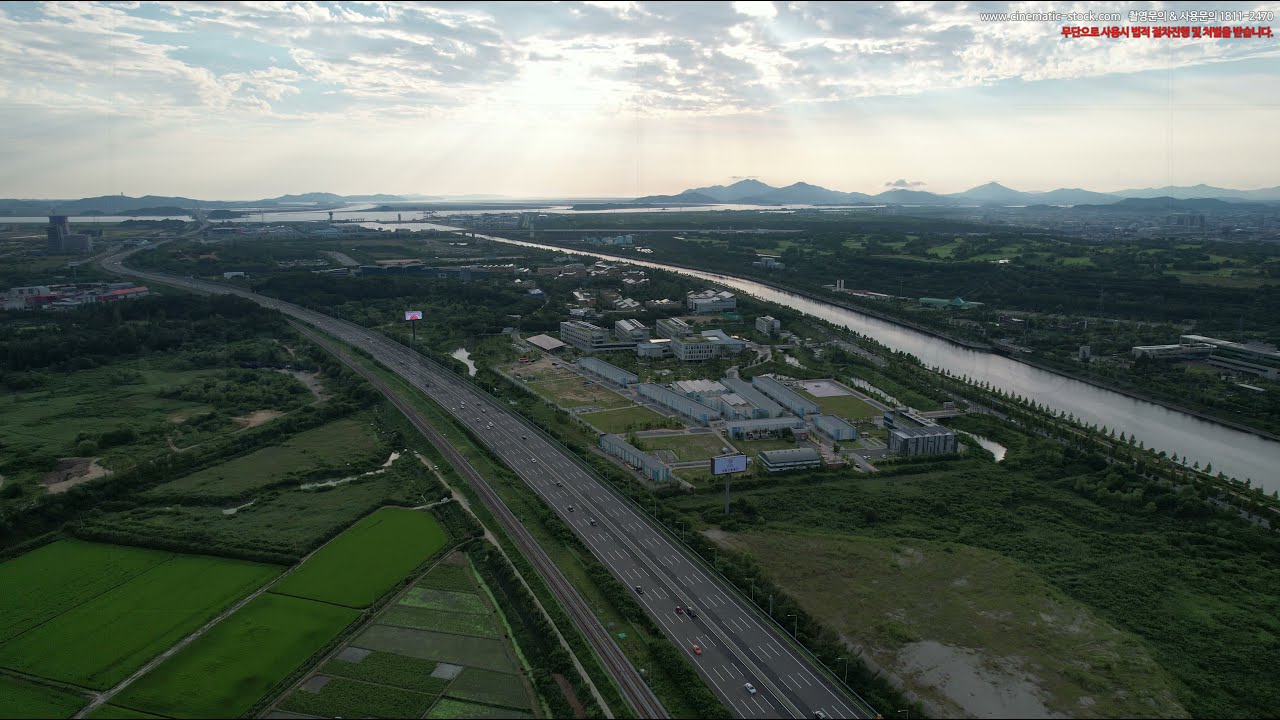The image captures an aerial view of a diverse landscape featuring a mix of natural and urban elements. Central to the image is a series of gray, industrial-looking buildings situated between a highway and a thin river that winds through the scene. To the left of the highway, expanses of farmland and various fields stretch out, punctuated by patches of trees and green vegetation. To the right of the river, more fields and trees are visible, along with a few scattered buildings. In the background, a range of mountains frames the skyline, with rays of sunlight piercing through the clouds, casting a dramatic light across the landscape. Cars on the highway appear tiny, indicating the photograph was taken from a significant height, possibly by a drone or an airplane. The image's color palette is primarily composed of greens and grays, with hints of blue and white. Additionally, there is text in the upper right corner that reads "cinematicstock.com" alongside some white and red Korean text.